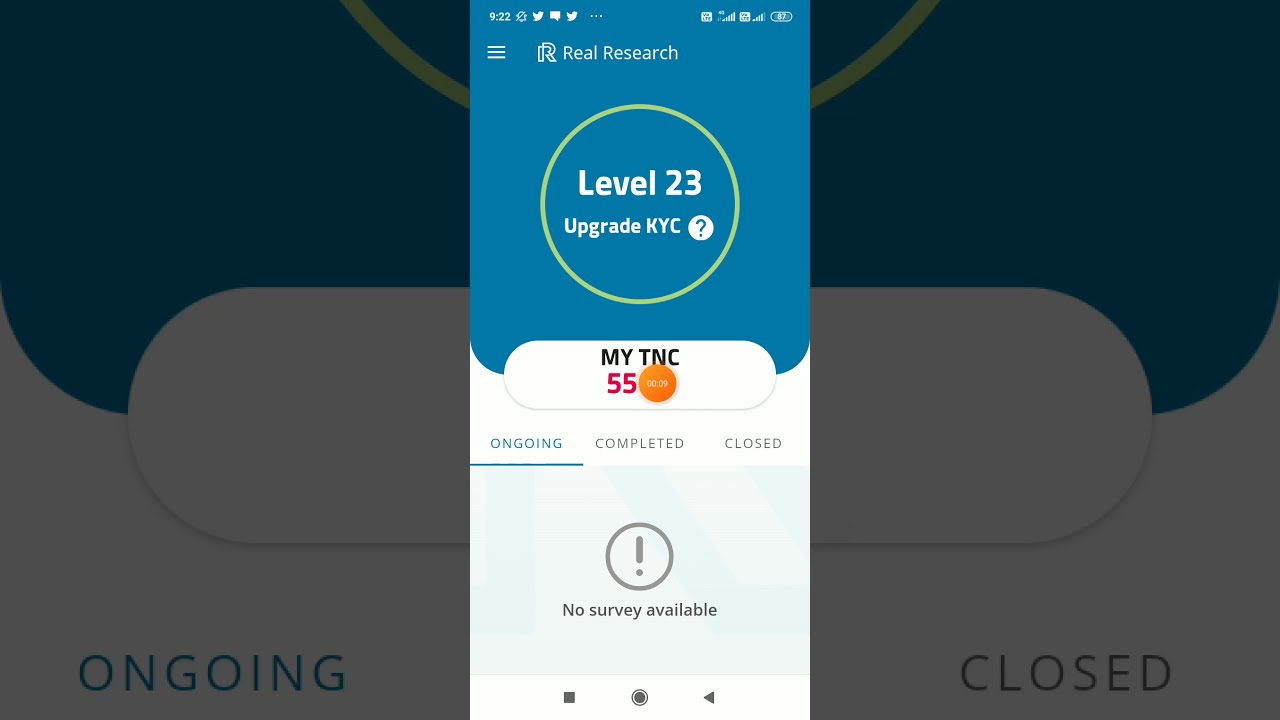The image depicts a screenshot of an app interface. At the very top, various icons are visible, including the time (9:22), battery level, cell signal, and notifications—two Twitter messages and a text message—alongside a "Do Not Disturb" icon. The app's title, "Real Research," is written in white text. Below the title, a green circular progress bar surrounds a white circle with a blue question mark, and inside this circle, white text reads "Level 23, Upgrade KYC." Beneath this, "My TNC" is displayed in black capital letters, followed by the number "55" in red. Further down, there are three tabs labeled "Ongoing," "Completed," and "Closed," with the "Ongoing" tab selected. Below the tabs, amid a gray background, there is a circle with a gray exclamation point and the message "No Survey Available." At the bottom, three symbols—square, circle, and sideways triangle—are arranged in white.